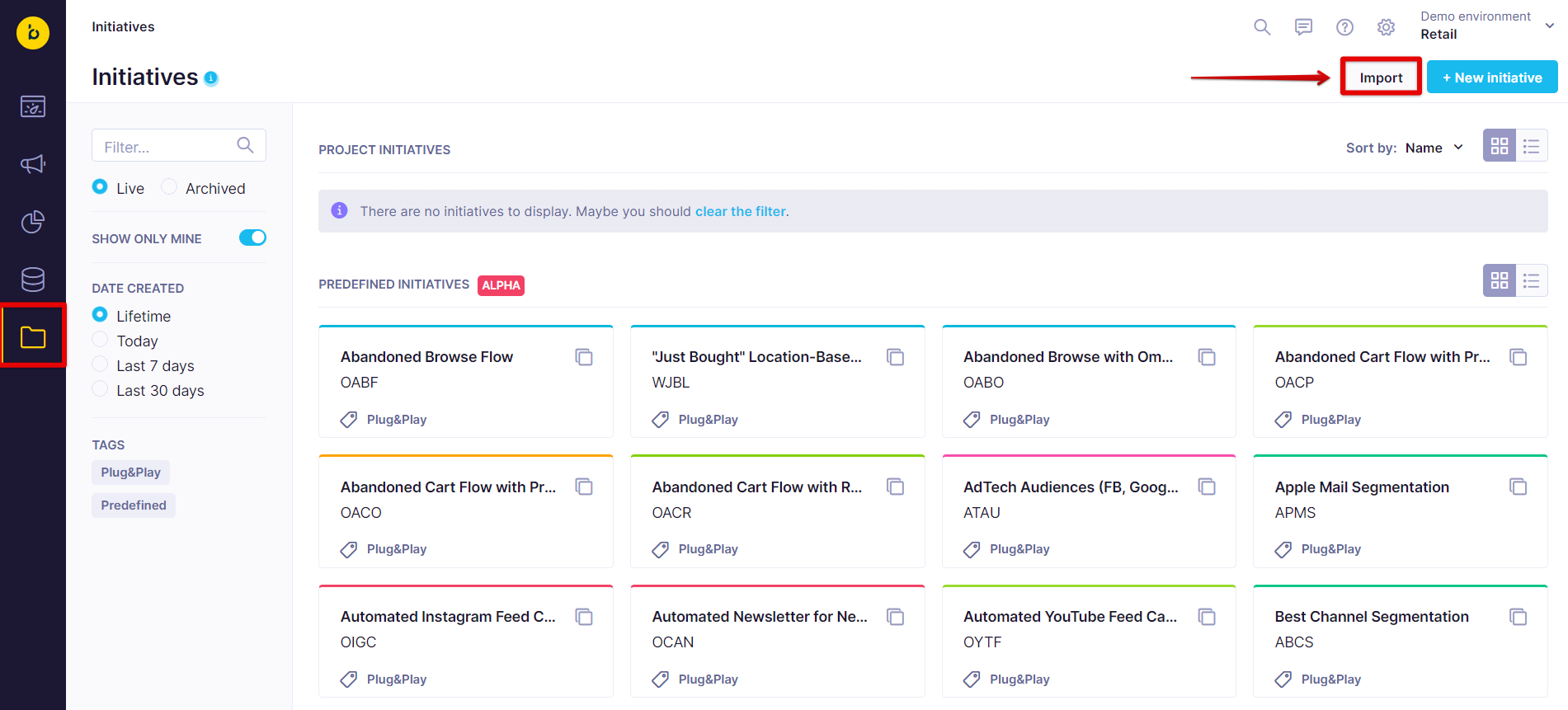The image portrays a partial computer screen, predominantly white, with a black vertical bar on the left-hand side, indicating an online platform interface. At the top of this screen, faintly visible words read 'Demo Environment,' with the word 'Retail' bolded directly beneath it. On the black sidebar, several icons are discernible: a yellow circle featuring a stylized letter 'B,' presumably the company logo, followed by icons resembling a calendar or folder, a speaker or sound symbol, a segmented circle, three stacked coins, and another folder icon.

In the white section, the word 'Initiatives' appears prominently at the top, accompanied by a search bar with filtering options. The main content area is titled 'Project Initiatives,' featuring a list of 12 sections with titles like 'Abandoned Browse Flow,' 'Abandoned Cart Flow,' and 'Best Channel Segmentation,' among others. This detailed visual layout suggests an organized interface for managing retail project initiatives.